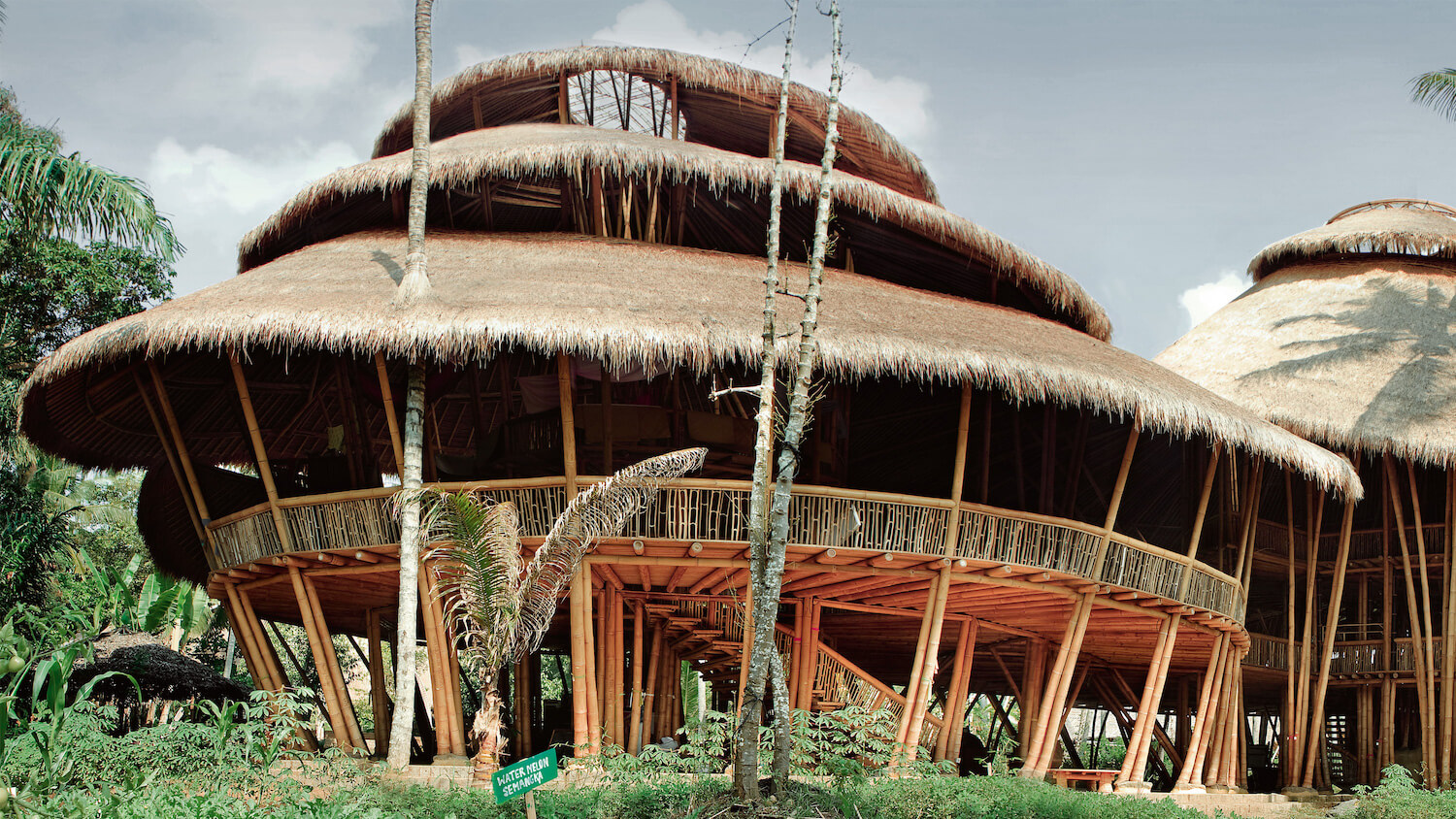The photograph captures a large, circular, multi-story structure situated in a lush, tropical jungle. This impressive edifice resembles a traditional hut but on a grand scale and is elevated off the ground, likely to avoid flooding. Built primarily from bamboo and wooden poles, including entire trees, the structure boasts a three-tiered thatched roof composed of what appears to be palm leaves and short vines, providing robust insulation. Each of the four levels, including the ground level, is open and airy, surrounded by railings that offer panoramic views of the vibrant, green foliage encompassing the site. The building's overall aesthetic and sturdiness suggest it serves as a communal gathering place. A stairway with a handrail leads up to the first floor, enhancing accessibility. The backdrop features an abundance of tropical plants, including palm and banana trees, under a clear blue sky dotted with clouds. A second, similar structure can be seen to the right, reinforcing the cohesive design and purpose of the complex. There is also an unreadable green sign in the foreground, the first word of which is "water," hinting at the presence of nearby amenities.